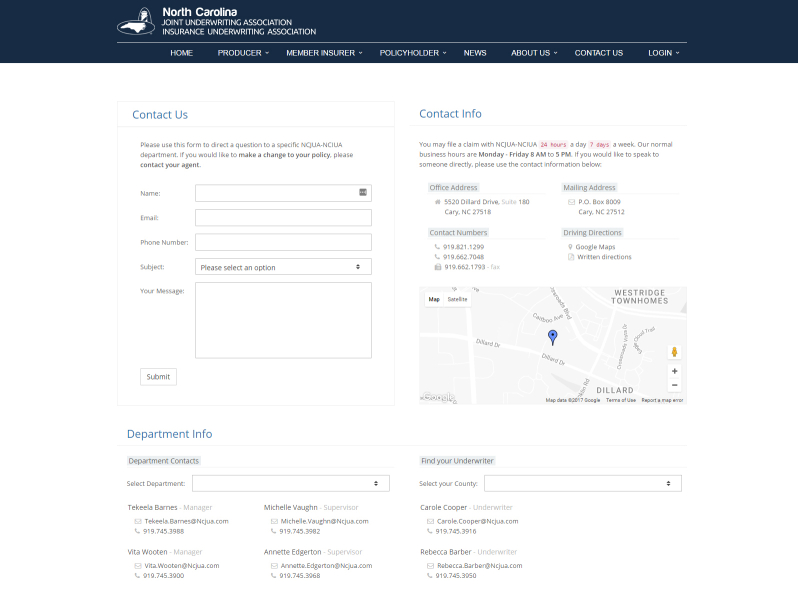The website for the North Carolina Joint Underwriting Association and North Carolina Insurance Underwriting Association features a clean, professional design with key navigational elements at the top and detailed contact options below. 

At the very top, a black header spans the width of the page, prominently displaying the organization's name "North Carolina Joint Underwriting Association Insurance Underwriting Association" in white text. To the left, an image of a duck adds a unique visual touch. The main navigation bar lies just below the header, presenting options titled "Home," "Producer," "Member," "Policyholder," "News," "About Us," "Contact Us," and "Log In."

Under this navigation bar, there is a "Contact Us" section. This section includes a form where users can enter their name, email, phone number, select a subject from a dropdown menu, type a message, and submit the form. To the right of this form, the website provides detailed contact information for their office, including the office address, mailing address, contact numbers, and a link for driving directions and further contact info. This information is highlighted at the top in blue, accompanied by a map with a single pin marking the office location.

Further down on the left-hand side, there is a "Department Info" section. This allows users to select their department from a list, complete with names, phone numbers, and email addresses for various contacts. Adjacent to this, a "Find Your Underwriter" section enables users to select their county and view information for underwriters such as Carol and Rebecca, along with their respective contact details for further inquiries.